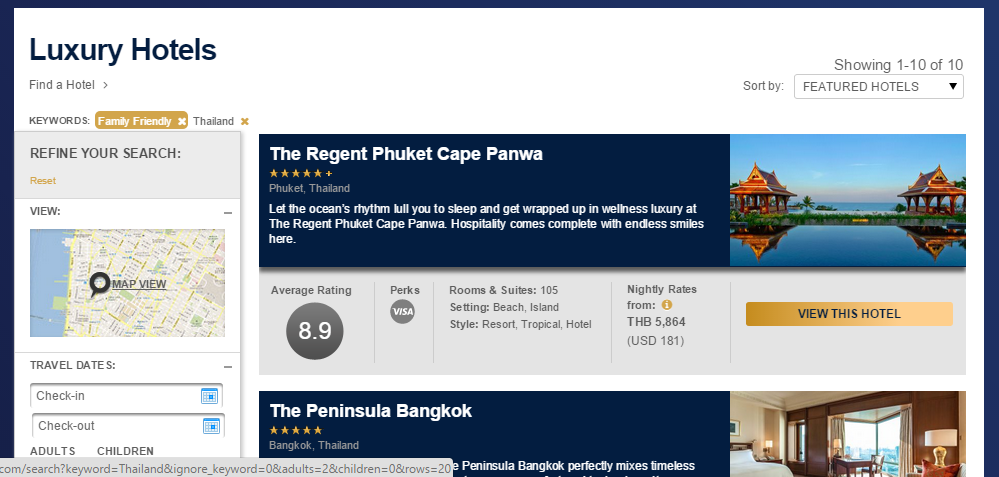Here is a cleaned-up and detailed descriptive caption based on the provided voice input:

---

Screenshot of a luxury hotel booking website featuring various accommodation options. At the very top left corner, the site lists "Luxury Hotels" as the main category, with an option to "Find a Hotel" just underneath. The page is also focused on keywords like "family-friendly" and "Thailand," helping users refine their search.

The left column, titled "Refine Your Search," offers multiple filters to narrow down hotel options. At the top of this column, users can reset their filters or view the map using a small map icon. Below, there are sections to input travel dates, specifying check-in and check-out times, as well as the number of adults and children traveling.

On the right side of this left column, the available hotel listings are displayed. The very top right corner of the page indicates that 10 hotels are being shown, with sorting options available through a dropdown bar currently set to "Featured Hotels."

The first hotel listing showcases the "Regent Phuket, Cape Panwa," a 5-star hotel located in Phuket, Thailand. It invites guests to be lulled to sleep by the ocean's rhythm and immerse themselves in wellness luxury. The description highlights the infinite hospitality, stunning beach, island-style resort, and tropical hotel settings. Accompanied by an image of the hotel, the listing notes an average rating of 8.9, various perks, a total of 105 rooms and suites, and nightly rates starting at THB 5,864. A call-to-action button encourages users to "View this hotel."

---